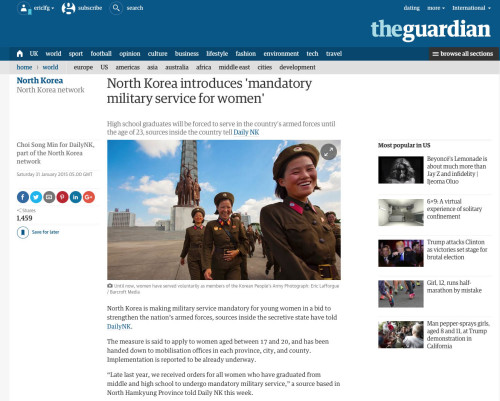The screenshot captures a web page from The Guardian newspaper. The page has a prominent blue frame running horizontally along the top, with "The Guardian" written on the right side. The main body of the page features a white background, dominated by a large central image. This image depicts female North Korean soldiers, with three women in the foreground wearing dark brown North Korean military uniforms, smiling as they walk. The background of the image showcases a bright blue sky dotted with white clouds. Above the picture, on the right side, the headline in black text reads, "North Korea introduces mandatory military service for women." To the left of the headline, in blue text, it says, "North Korea." This detailed composition of the page offers a vivid visual and contextual glimpse into the article's focus on North Korea's new policy for women in the military.